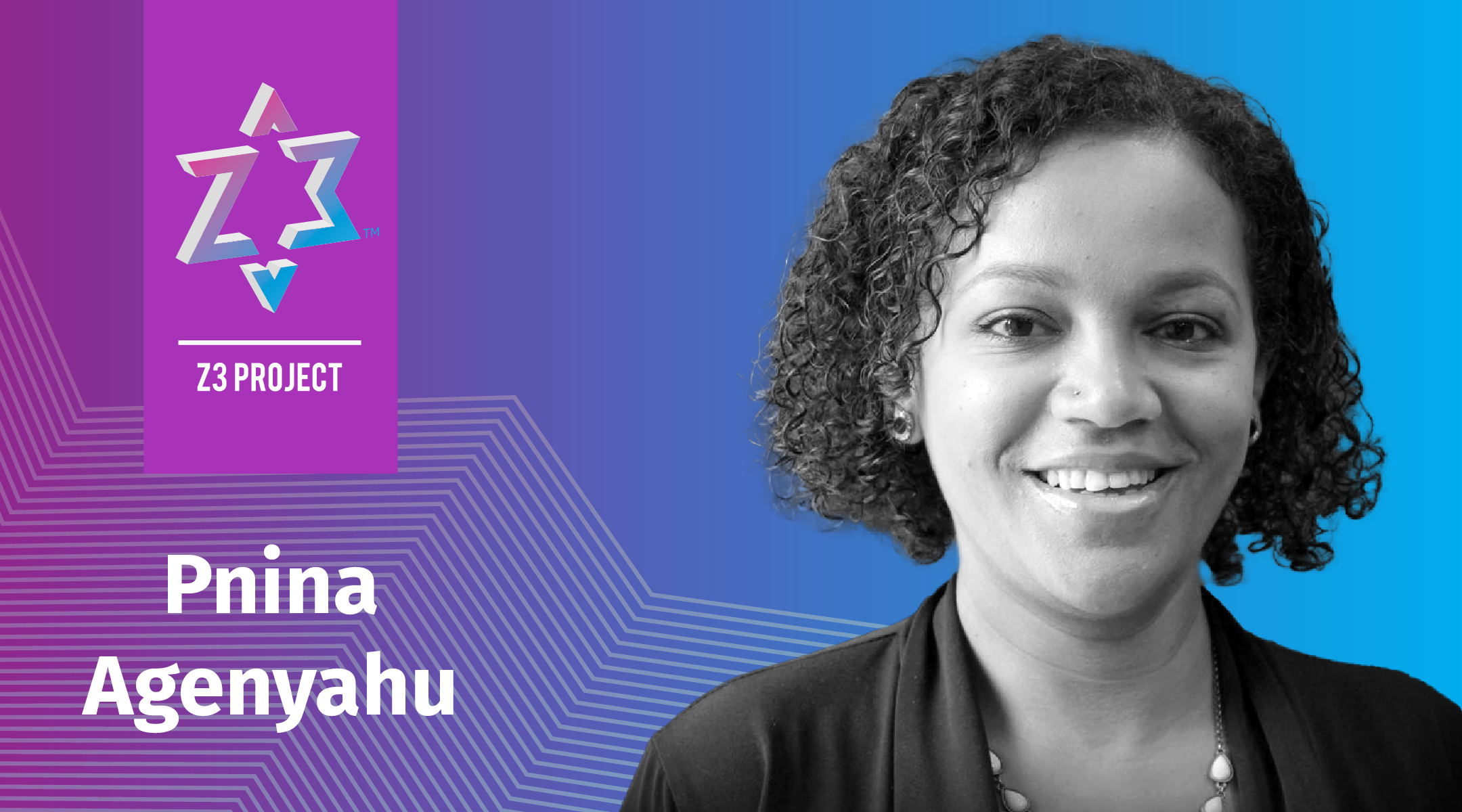This marketing photograph, set in a horizontal, rectangular orientation, features a smiling young black woman in her 20s positioned on the right side. She has short, curly black hair that is parted on the left and falls slightly over her forehead to the right. Her contemporary outfit consists of a black jacket paired with a beaded necklace. The image is rendered in black and white, enhancing her bright, cheerful expression.

The background of the photograph transitions smoothly from a bright blue on the right to a darker bluish-purple hue, further evolving into a magenta pink on the far left. This gradient is interrupted in the upper left corner by a vertical, bright magenta banner. Within this banner, a logo displaying the characters "Z" and "3" arranged horizontally side-by-side forms a shape resembling the Star of David. Below this geometric emblem, a horizontal white line separates the logo from white, uppercase text reading "Z3 PROJECT." Further down, a white polygon graphic serves as a backdrop to the name "P. Nina Agenyahu," written in white lettering, spanning two lines.

White spiral designs subtly decorate the gradient background, adding an intriguing layer of visual interest to the composition. This thoughtful arrangement makes the photograph suitable for a professional profile on digital social media or a polished presentation.